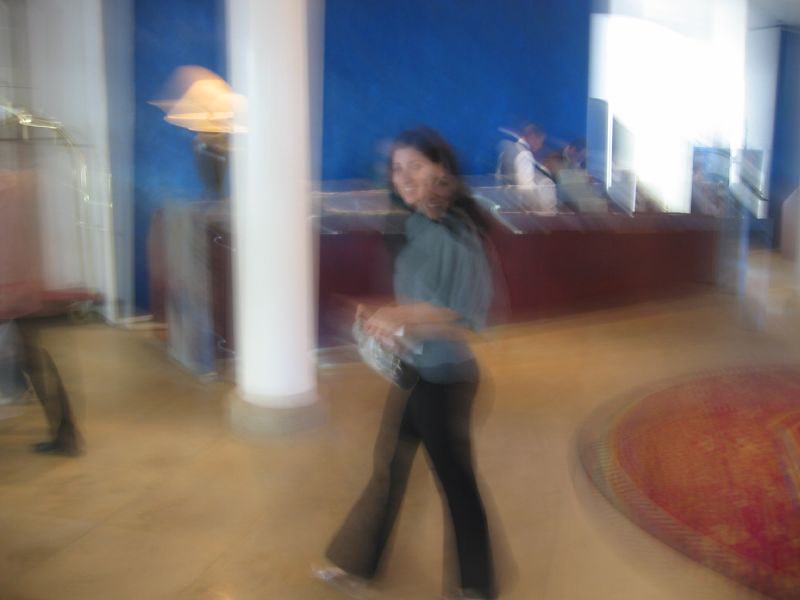The image depicts a blurry photograph, likely taken in motion, of a woman walking through what appears to be a hotel lobby. The lobby's floor is light brown, complemented by a large, circular Persian-style rug in predominantly red and yellow hues located to the right of the frame. In the foreground, the woman has long black hair just past her shoulders and is smiling directly at the camera. She is attired in black dress pants, a light gray short-sleeved sweater, and silver high-heeled sandals. She is carrying a pale whitish or silver bag. Behind her, slightly reflected due to the blurriness, is a porter carrying her luggage, visible through the back leg and blue suitcases he’s handling. The reception area features a long mahogany brown desk with three hotel staff members engaged in conversation, likely addressing a matter of interest. The backdrop includes a prominent blue wall and to the left, a large white support column. A lamp with a white lampshade is positioned at the end of the desk. Altogether, the scene captures a bustling moment within the elegant hotel lobby.